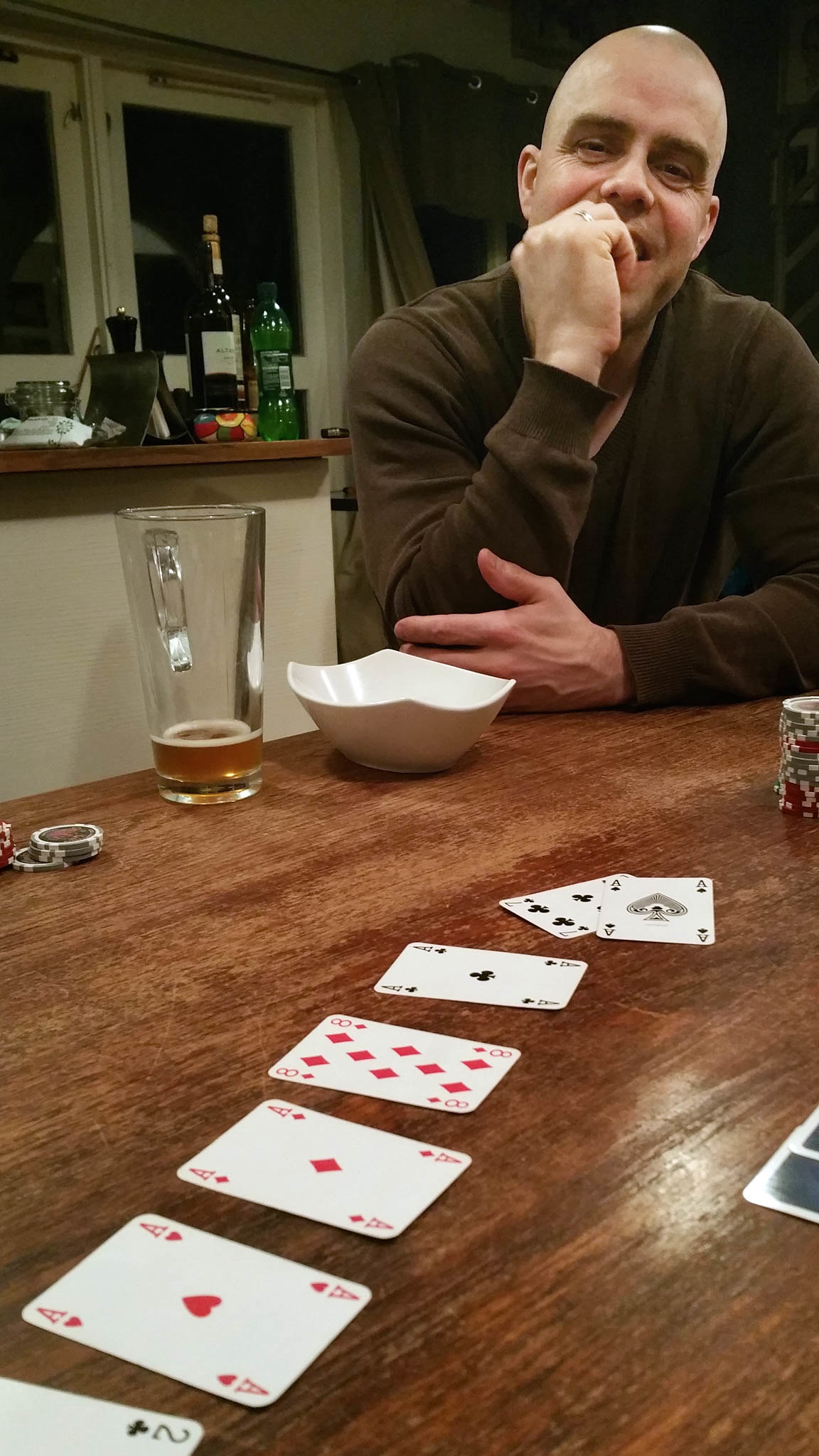In this image, a lively card game is taking place at an angled, woodgrain table. Seated at the top right corner is a bald man, who appears to be smiling with his hand up by his mouth. He wears a brown shirt and likely has dark eyes. In front of him sits a uniquely shaped bowl with pointed edges curving upwards, and to its left is a glass pitcher of beer, containing only about an inch and a half of liquid.

Spread out on the table are several playing cards. In the left-hand corner, there is a two of clubs, followed by an ace of hearts, an ace of diamonds, an eight of diamonds, and an ace of clubs. Closer to the man are additional cards, including an ace of spades and a four of clubs. To the far right, a deck of cards lies face down, concealing the remaining cards.

The background features an assortment of wine bottles, a window, and a shelf filled with various items, adding to the cozy, intimate ambiance of the scene.